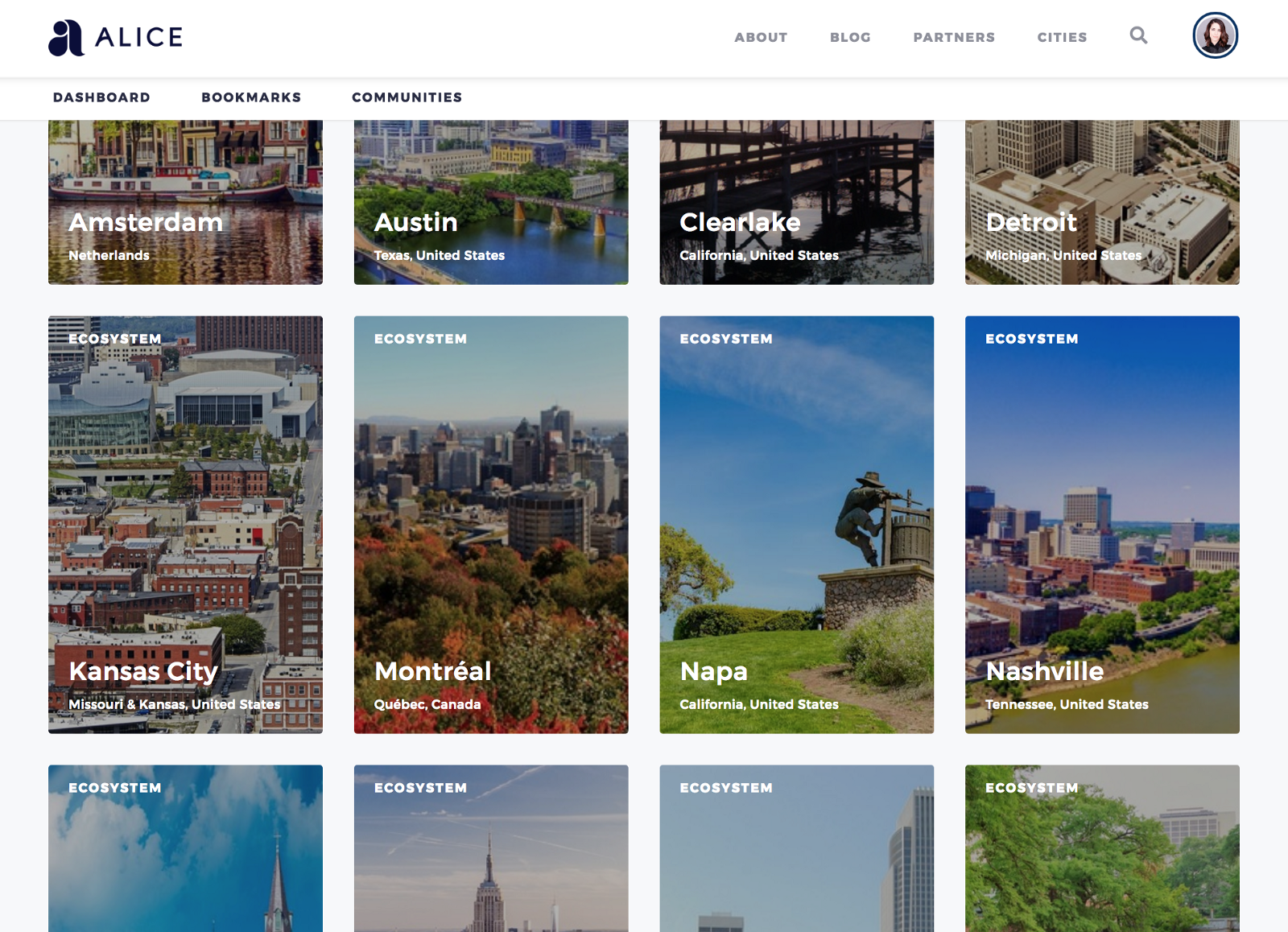The image is a detailed screenshot of a web page featuring three rows of photographs, with two full rows and part of a third visible. The background at the top is white. In the upper-right corner, gray font in capital letters reads "ALICE," adjacent to a large, stylized lowercase 'a,' presumably the company logo. To the right are menu items in light gray font: About, Blog, Partners, and Cities, accompanied by a small search icon. In the upper-right corner is a tiny profile photo of a white woman with brown hair.

To the left, beneath "Alice," are additional menu options: Dashboard, Bookmarks, and Communities. The top row showcases four photos overlaid with city names in white font: Amsterdam, Austin, Clear Lake, and Detroit, each displaying a cityscape view. The second row contains larger, vertical rectangle photos labeled Kansas City, Montreal, Napa, and Nashville. These depict varied scenes: Napa's lush green landscape under a blue sky, Nashville's distant city view with a blue sky, and Montreal's aerial view of an autumnal park with vibrant fall colors.

The bottom row is partially visible, revealing only the upper sections of some photos—primarily skies in various shades, from bright blue to slate gray-blue, with hints of treetops, but no city names.